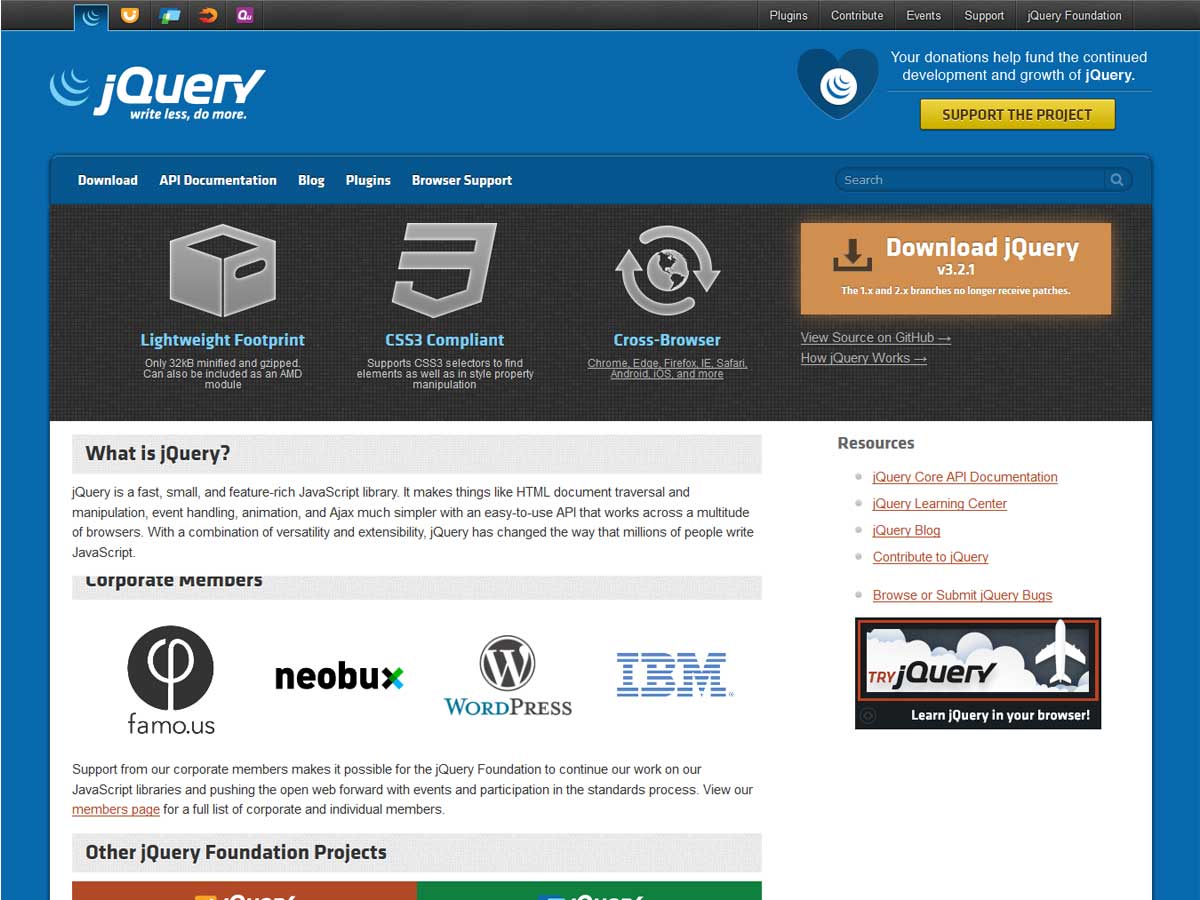A detailed descriptive caption for the provided image of the webpage could be:

---

This is a screenshot of an outdated jQuery webpage. The header showcases an old Mozilla Firefox logo, suggestive of the site's age. Key navigation links at the top include "Plugins," "Contribute," "Events," "Support," "Query Information," and "Foundation." Below the header, a yellow rectangular banner reads, "Your donations help fund the continued development and growth of jQuery. Support the project." Further down, the webpage offers various options: "Download," "API Documentation," "Blog," "Plugins," and "Browser Support." Prominently in bright orange, there is a link to "Download jQuery version 3.2.1," followed by additional links, including "View Source on GitHub" and "How jQuery Works." Another highlighted section, possibly in a square box, invites users to "Try jQuery" and "Learn jQuery in your browser." Five underlined resources are listed beneath the heading "What is jQuery?" The section on corporate members acknowledges "famo.us," "NeoBUX," "WordPress," and "IBM" as contributing organizations, with "jQuery Foundation Projects" being mentioned alongside text emphasized in red and green.

---

This caption provides a comprehensive and structured description of the image, making it clear and informative.